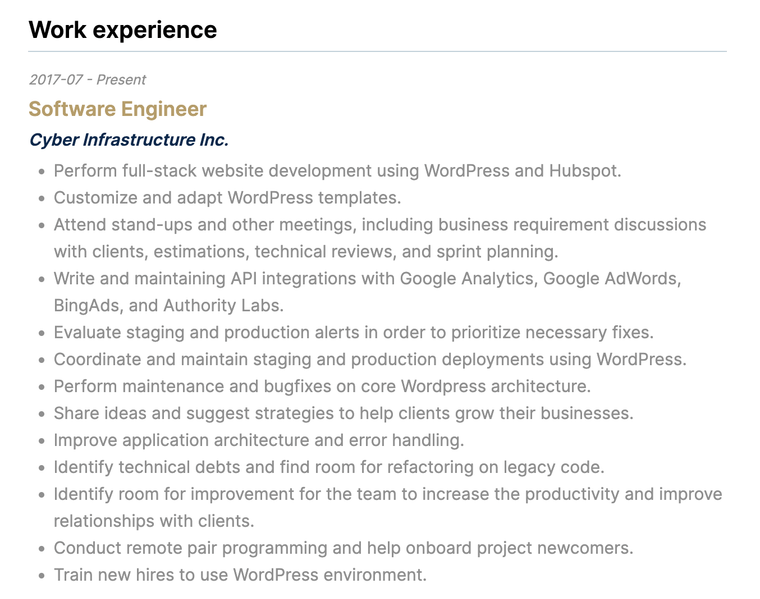**Work Experience**

---

*2017-07 - Present*

**Software Engineer**

**Cyber Infrastructure Inc.**

- Perform full-stack website development using WordPress and HubSpot.
- Customize and adapt WordPress templates.
- Attend stand-ups and other meetings, including business requirement discussions with clients, estimations, technical reviews, and sprint planning.
- Write and maintain API integrations with Google Analytics, Google AdWords, Bing Ads, and Authority Labs.
- Evaluate staging and production alerts to prioritize necessary fixes.
- Coordinate and maintain staging and production deployment using WordPress.
- Perform maintenance and bug fixes on core WordPress architecture.
- Share ideas and suggest strategies to help clients grow their businesses.
- Improve application architecture and error handling.
- Identify technical debts and find opportunities for refactoring legacy code.
- Identify areas for team improvement to increase productivity and enhance client relationships.
- Conduct remote pair programming and help onboard project newcomers.
- Train new hires to use the WordPress environment.

All bullet points are written in gray.